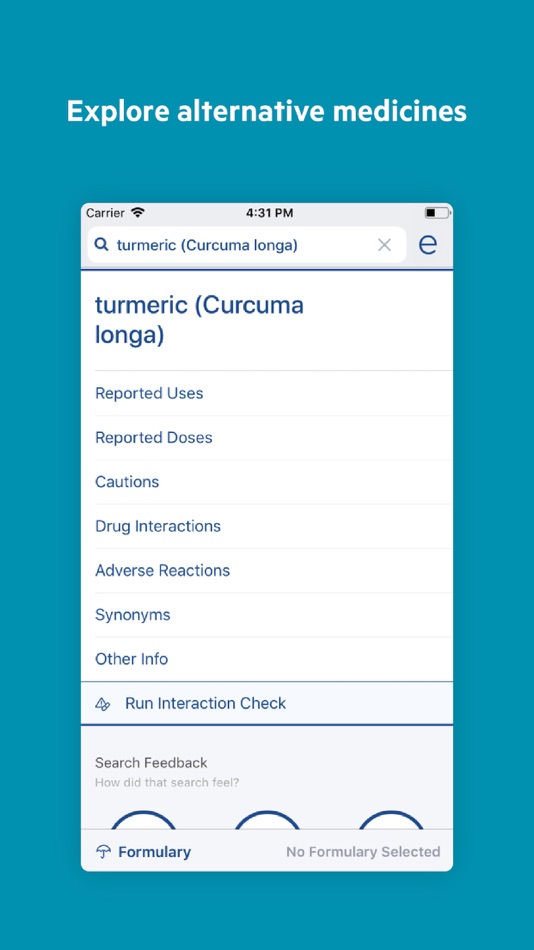The image features a light blue background with the title "Explore Alternative Medicines" prominently displayed at the top in white letters. Just below the title, there is a white rectangular box showing "Carrier, 4:31 PM," with an icon indicating about one-third of battery life remaining. Beneath this, there is a search box with "Turmeric Curcuma Longa" entered into it. 

Directly below the search box, in larger font, the term "Turmeric Curcuma Longa" is again displayed. Following this are various informational categories: "Reported Uses," "Reported Doses," "Cautions," "Drug Interactions," "Adverse Reactions," "Synonyms," "Other Info," and an option to "Run Interaction Check." 

Further down, there is a section titled "Search Feedback" asking, "How did that search feel?" Below this, the term "Formulary" is listed, with "No Formulary Selected" noted to its right. Additionally, three bent lines appear just above these features, likely representing an icon or symbol related to the interface.